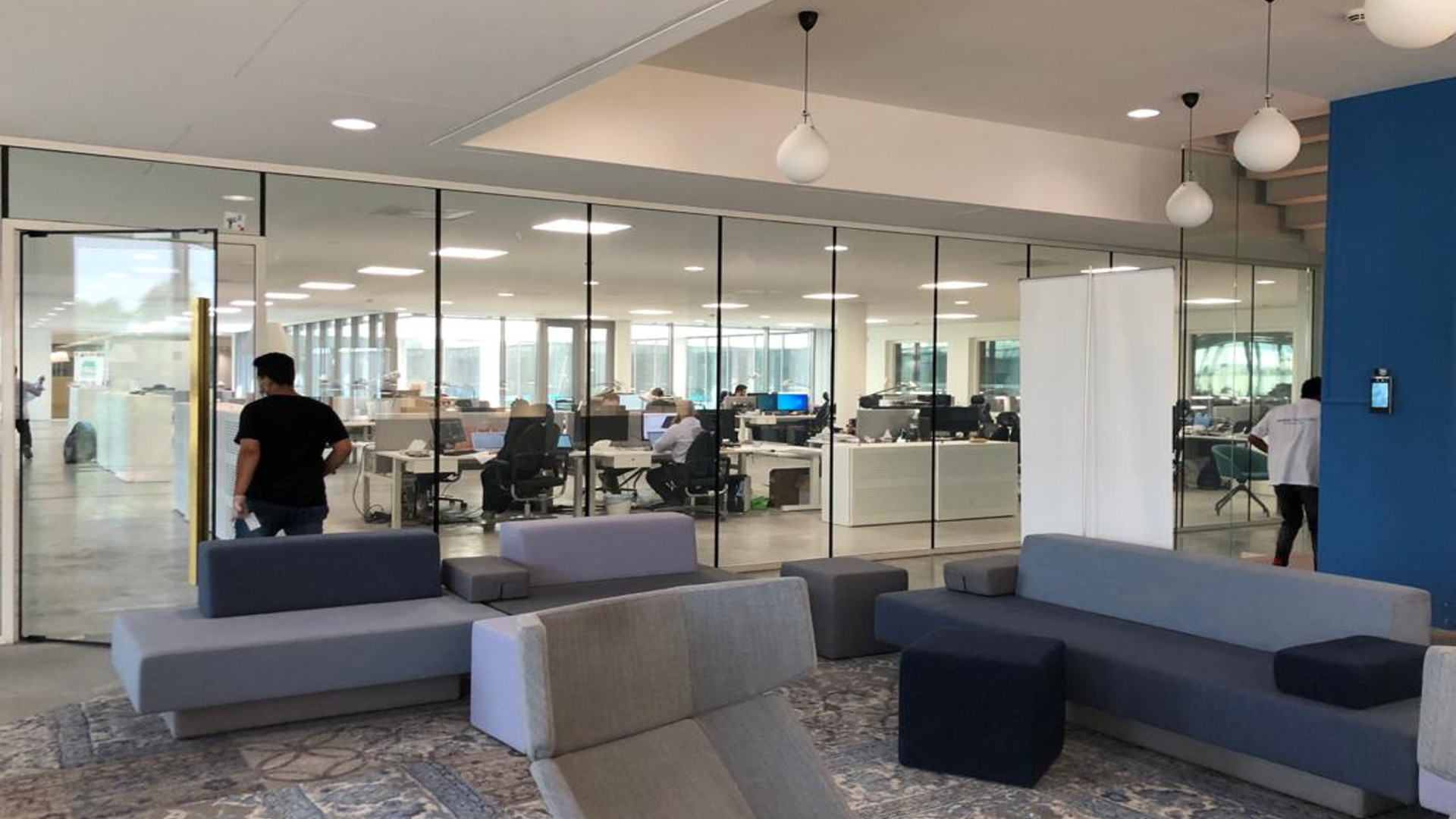In the reception area of a large, modern office building, visitors are greeted by sleek, contemporary furniture upholstered in shades of blue, gray, and violet. Although the seating appears stylish, it may not provide optimal comfort for those waiting. The area is well-lit, with modern light fixtures hanging from the ceiling, adding to the sophisticated ambiance.

Just beyond the reception area, a transparent glass wall offers a view into the bustling open workspace. Rows of employees are stationed at desks, their backs turned towards the reception area, focusing on their computer screens. Although this layout allows supervisors to easily oversee the workspace, the visibility of the screens raises concerns about data security, particularly in a space frequented by visitors.

The expansive office area is carpeted, and natural light floods in from large windows, creating a bright and inviting environment. The workspace is arranged in an open plan, with clusters of desks interspersed by occasional stations, fostering a collaborative atmosphere. The overall design promotes a sense of openness and community among the employees.

In the midst of this scene, a man appears ready to enter through a glass door, while another person walks by, contributing to the dynamic and busy feel of the environment. Despite the potential security trade-offs, the office's light-filled, airy design likely offers an appealing workspace for its occupants, particularly on sunny days.